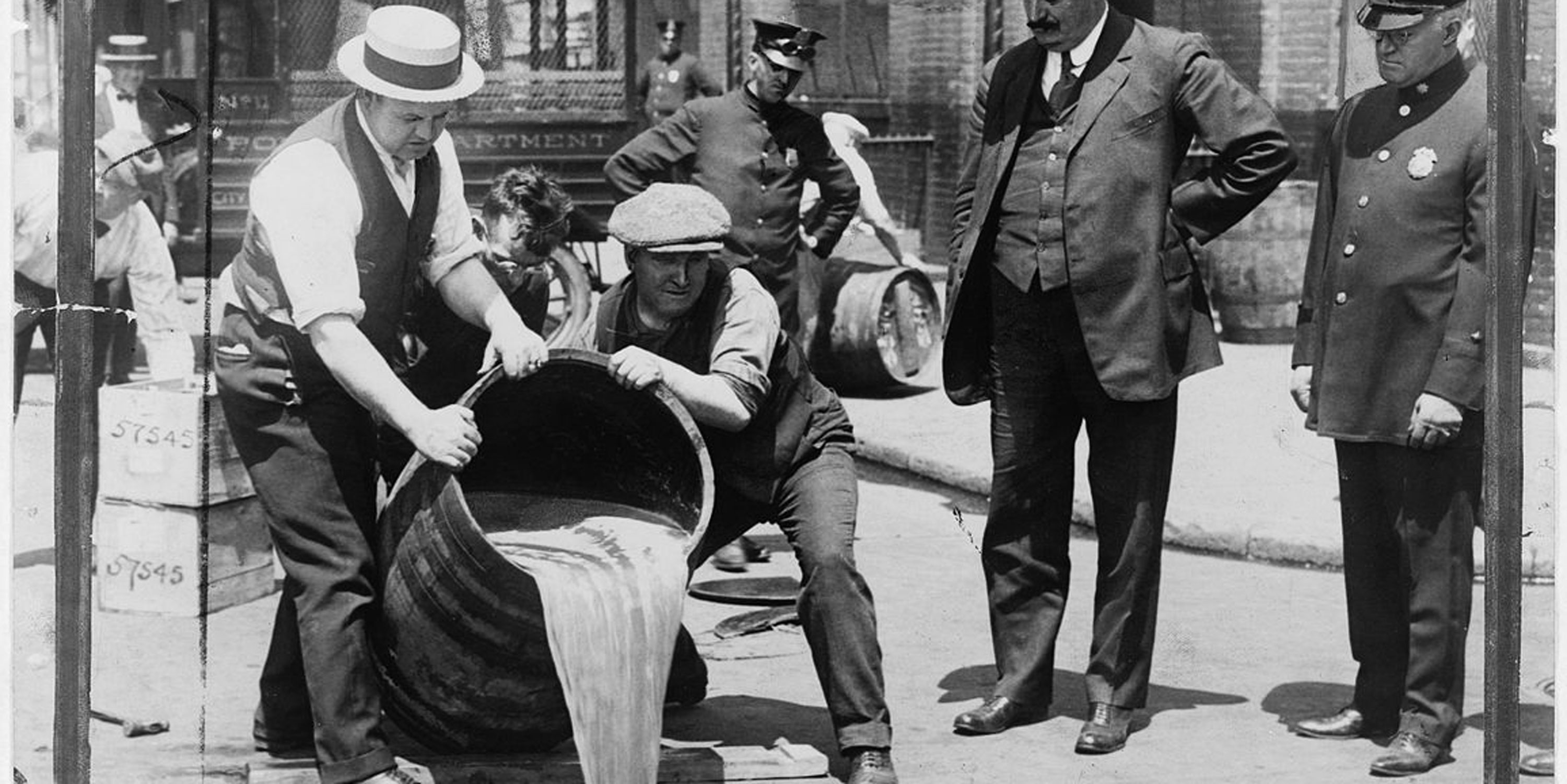This vintage black-and-white photograph captures a lively street scene outside a police department building. In the foreground, two men are dousing the street with a cloudy, foamy liquid from a wooden barrel, presumably beer or ale. The man on the left, dressed in a rolled-up white shirt, dark vest, and black pants, is leaning over with both hands atop the barrel. His companion, positioned squatting to the right of the barrel and facing the camera, wears a short-sleeved shirt, black pants, and a hat. Behind these two men, a police officer with hands on hips and dressed in a blue shirt and hat observes the proceedings closely, appearing slightly annoyed. To their right stands a partially visible man in a three-piece suit with his left hand on his hip, facing the camera with a slightly turned stance. Adjacent to him, an older policeman with white hair, glasses, and a black button-up jacket also watches the scene intently. The background is dotted with more policemen and onlookers, partially obscured by the building labeled "Police Department." This bustling tableau portrays a moment of enforcement, likely during a prohibition-era crackdown, with crates stacked nearby adding to the evidence of a possibly larger operation underway.